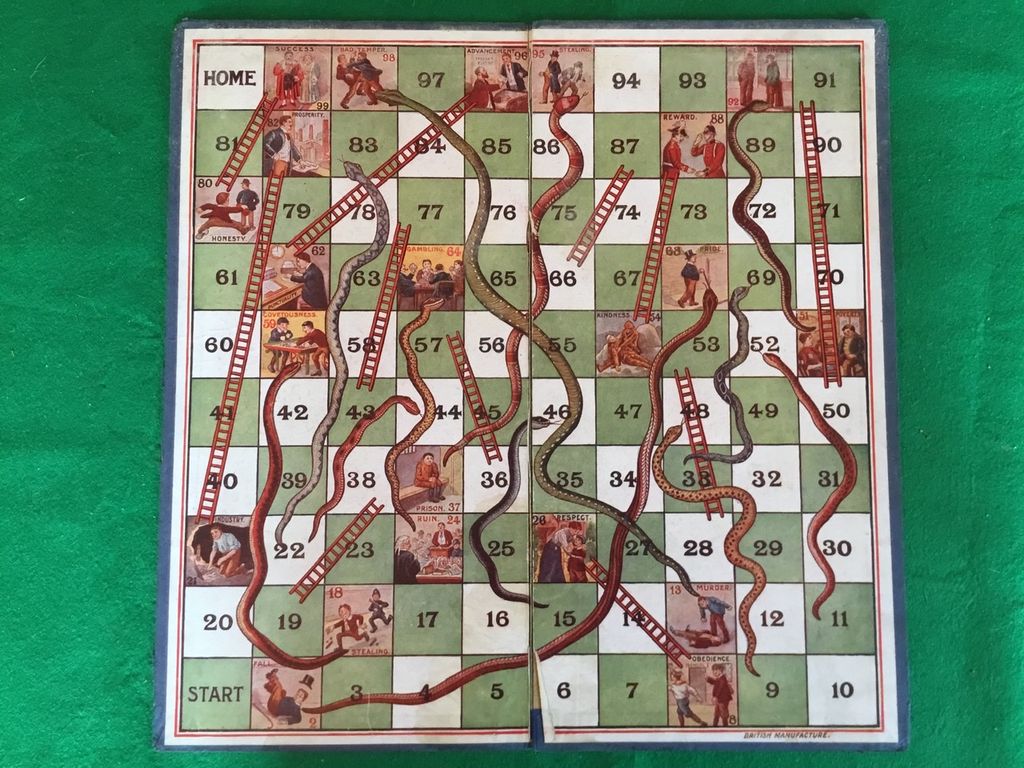The image depicts a well-worn, tattered board game of Snakes and Ladders, laid out on a green surface. The board's edges are blue, surrounding a 10x10 grid of 100 numbered squares. The squares alternate between green and white, beginning with 'Start' at the bottom left, numbered 1, and ending with 'Home' at the top left, numbered 100. Intricate illustrations on the squares depict various activities and virtues, including children running, laughing, playing in the snow, and sitting at a table. The game features numerous brown ladders and serpentine snakes that create a complex path across the board. Landing on a ladder's base allows players to advance to its top, while landing on a snake's head forces them to descend to its tail, embodying a moral lesson within the gameplay. The board's appearance shows signs of age, with faded colors and some rips where it folds.